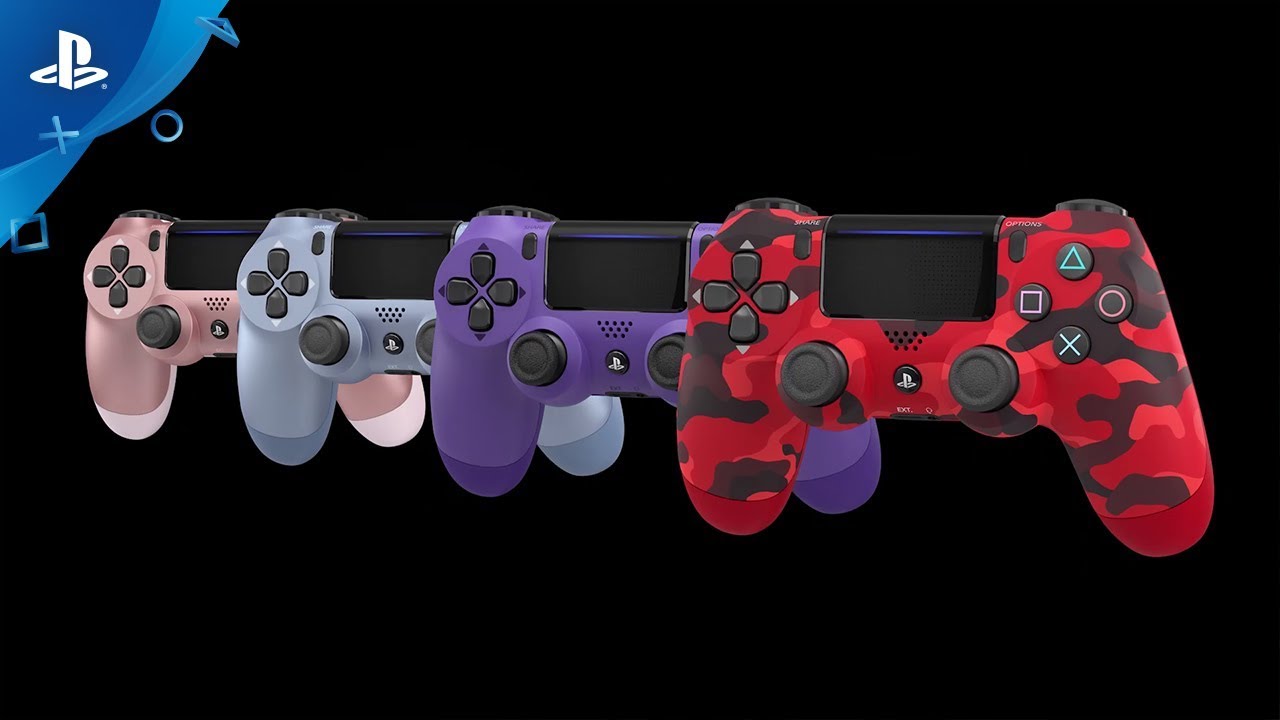The image features four PlayStation controllers displayed against a flat black background. In the top left corner, there is a triangular dark and light blue banner with the PlayStation logo in white. The four controllers, positioned across the center of the image, are overlapping slightly and showcase a variety of colors. The colors include a dusty tan, a robin's egg blue with a possible frosted finish, a violet, and a distinctive red camouflage print with black highlights. The controllers, likely from the PlayStation 4 series, exhibit a mix of solid and patterned designs, with the red camouflage one standing out due to its unique print. The image does not contain any explanatory text or additional graphical elements other than the PlayStation logo.